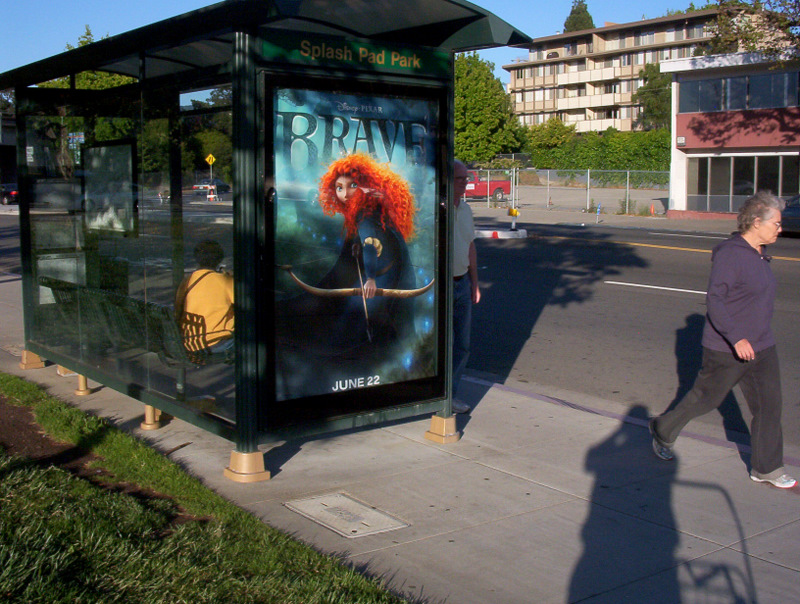The image captures a city street scene featuring a bus stop with a dark forest green frame and transparent glass panels enclosed on three sides. Prominently displayed on the bus stop is an advertisement for the Disney Pixar movie "Brave," showcasing a red-haired girl with a bow and arrow, with the release date June 22nd. The bus stop is also marked with a "Splash Pad Park" sign. 

Within the bus stop sits a person, likely female, dressed in a yellow sweatshirt and blue jeans. Walking past the bus stop are a couple of individuals: one is a man in a purple pullover and black pants, while another is an older gentleman in a white pullover and blue jeans. 

In the background across the city street, various buildings are visible, including a large one and a two-story structure with glass windows. Past these buildings, there's a parking lot. Additionally, a red building and a four-story apartment complex with balconies can be seen, along with a red truck parked behind a fence near some bushes. The city street intersects nearby, adding to the bustling urban atmosphere.